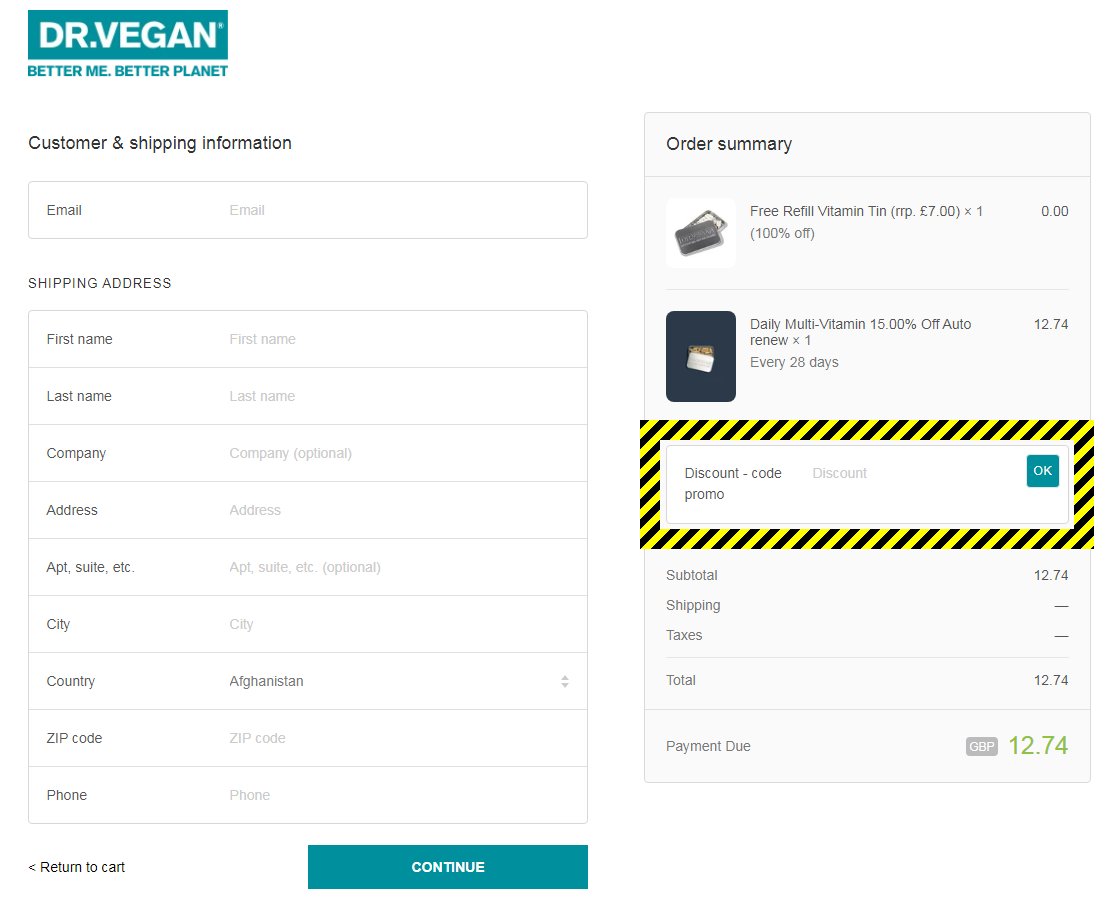This is an image of an order summary screen. 

In the top left corner, there is a teal box with white text that reads "Dr. Vegan," and below that, in the same teal text, it says, "Better Me. Better Planet." 

Underneath this, there is a section for customer and shipping information. There is a box labeled "Email" with light gray text indicating where to input information. To the right, there is space to type the email address. 

Following this, there is a line labeled "Shipping Address" with nine subsequent boxes for input. These are labeled in order: "First Name," "Last Name," "Company (Optional)," "Address," "Apt, Suite, etc.," "City," "Country (Afghanistan)," "Zip Code," and "Phone." Each box has placeholder text in light gray indicating the type of information needed, except for "Company" which includes the clarification "(Optional)." 

Below this section, there is a button labeled "Return to Cart" pointing to the left, and a "Continue" button with white text on a teal background.

On the right side, there is an order summary box that features an image of a vitamin tin. It lists "Free Refill Vitamin Tin MP7 x1" with a cost of $0.00, indicating it is 100% off. It also lists "Daily Multi-Item, 15% Off Auto Renew x1 every 28 days" with a price of $12.74. 

There is a red and black banner that reads "Discount Code Promo Discount." Below this is a teal button labeled "OK." 

The subtotal is shown as $12.74. Shipping costs are marked with a dash, indicating no charge at this time. Taxes are also indicated with a dash. The total amount due is $12.74, and at the bottom, it states, "Payment Due: GBP 12.74."